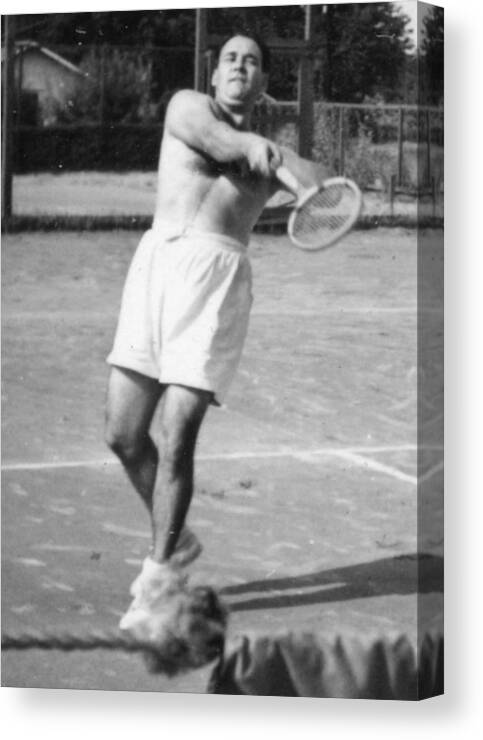The image is a black and white photograph printed on a canvas, giving it a slightly three-dimensional appearance, particularly on the right side. It captures a shirtless, muscular man in mid-swing, playing what appears to be tennis. He is wearing white, somewhat baggy shorts and white tennis shoes. His body is turned to the right, leaning back as he strikes the tennis ball with a racket that has a roundish net. In the background, a chain-link fence, a row of trees, and poles are visible. Additionally, there is a structure resembling a house or garage in the top left corner, along with some vegetation and possibly a brick fence. A rope with some fabric or a garment draped over it is situated at the bottom right of the image. The court he is playing on is marked with white lines, and his shadow is cast directly behind him, adding depth to the photograph.